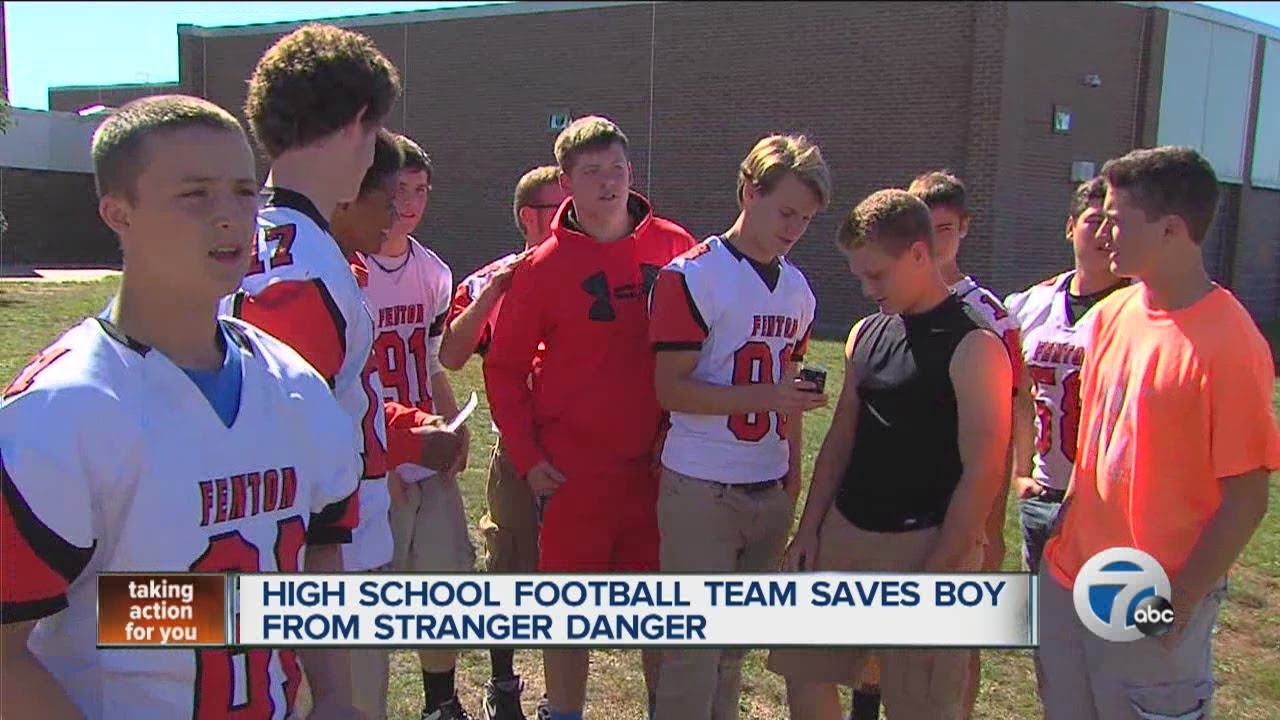This image from ABC Channel 7’s newscast "Taking Action For You" shows a group of high school football players from Fenton High School standing on a grassy field in bright daylight, with a clear sky overhead. The headline reads, "High School Football Team Saves Boy from Stranger Danger." The team, dressed in red, white, and black jerseys—some displaying numbers, such as 91, and names like Fenton—are gathered in what appears to be their school grounds. Among them, one boy in a sleeveless black shirt and tan shorts, possibly the boy who was saved, stands out. Another boy is seen holding up his cell phone, sharing something with a teammate. The school building is visible in the background, emphasizing that this heroic act occurred in their familiar turf. This special report highlights the team’s bravery in protecting a young boy from an unknown kidnapper, capturing a moment of community pride and awareness on the broadcast, known for its community-focused segments.